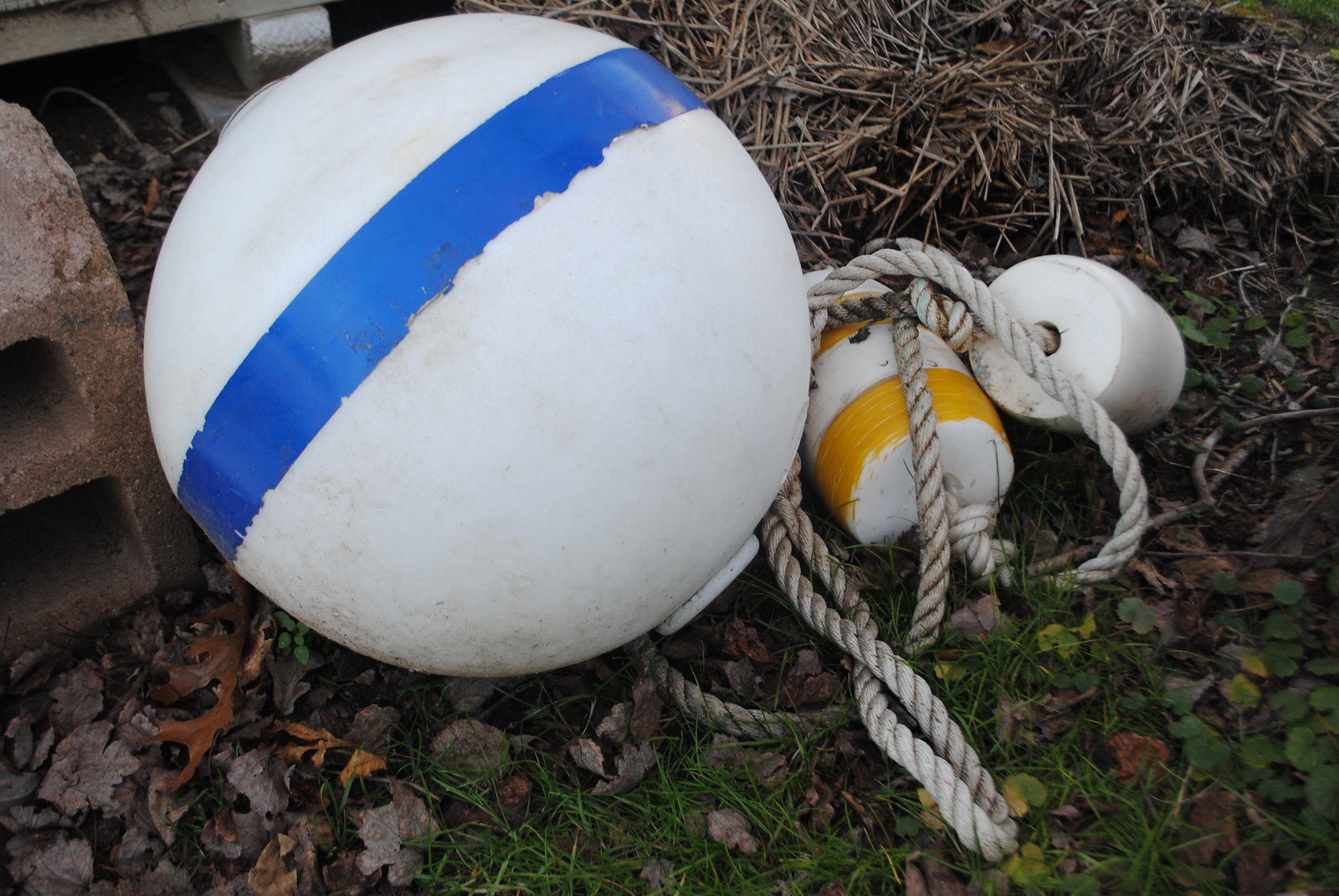In the photo, we see a scene featuring what appears to be marine equipment laid out on the ground. The central focus is a large, round, white buoy with a blue stripe around its circumference. Attached to this buoy is a white rope, which is visibly worn. Flanking the buoy are two smaller float-like objects: one is white with yellow stripes, while the other is solid white. These objects are also connected by the same white rope. The background consists of a mixture of dead leaves, brown grass, and patches of green grass, hinting at a possibly damp or dewy ground. To the left edge of the frame, part of a large, gray cement block is visible. In the background, there seems to be a pile of straw and some indistinct shapes, adding to the overall scene that suggests an outdoor storage area for marine gear.